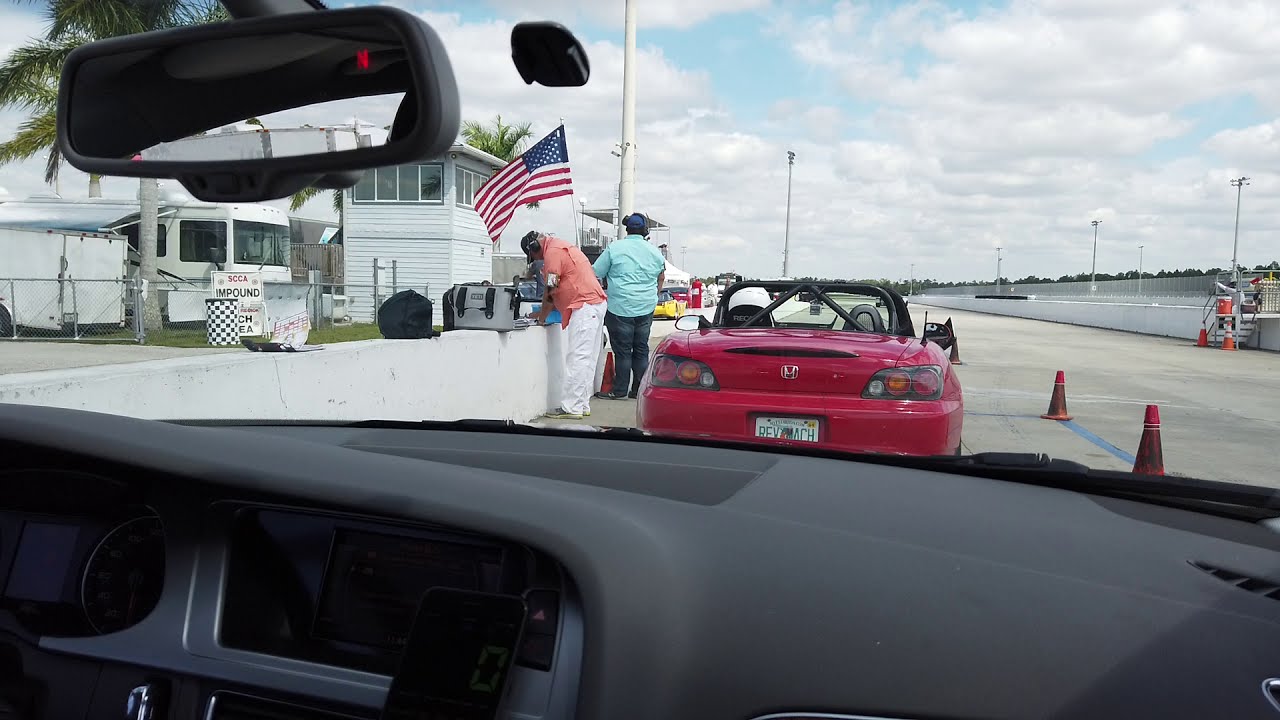The photograph appears to be taken from inside the passenger seat of a car, capturing a scene outside the windshield. In the foreground, the dashboard and rearview mirror are visible, with the latter positioned in the upper left-hand side of the image. Directly ahead, a red convertible sports car, identified as a Honda with a black roll bar and Florida license plate reading "REV MACH," is parked. To the right of the vehicle, two orange traffic cones are positioned on a cement surface. On the left side, two men stand in front of a short white wall; one wearing an orange shirt with white pants, and the other donning a teal shirt with jeans. An American flag is placed between the two individuals. Behind the wall, buildings are visible, with large light poles and a chain link fence in the distance suggesting a racetrack or event area, possibly for racing or NASCAR. The sky is a mix of blue with some clouds, and palm trees are seen in the background, indicating a likely Florida location.